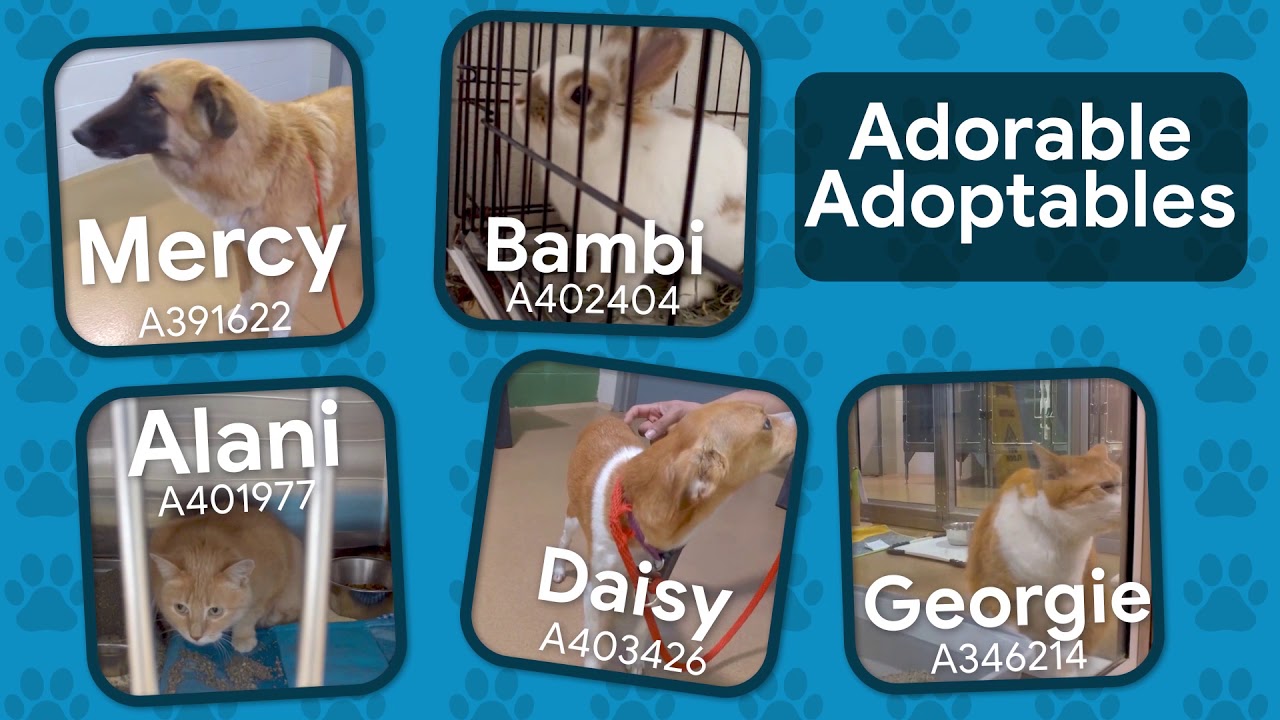This is a screenshot of a digital banner or webpage with a teal background adorned with paw prints, serving as colorful wallpaper. Centered on the page are five photographs of various animals up for adoption, each accompanied by their respective registration numbers. In the top right corner is a dark green sign with the text "Adorable Adoptables" written in white.

The featured animals are as follows:
1. Mercy, a dog with the registration number 8391622, located on the far left.
2. Bambi, a bunny in a cage, with the registration number A402404, positioned to Mercy's right.
3. Alani, a cat in a crate with the registration number A401977, situated on the second row from the left.
4. Daisy, a short-haired dog with a red leash and the registration number A403426, found to Alani's right.
5. Georgie, an orange and white two-toned tabby cat, with the registration number A346214, displayed on the far right.

This banner aims to highlight the adorable animals available for adoption, encouraging viewers to consider giving these pets a loving home.